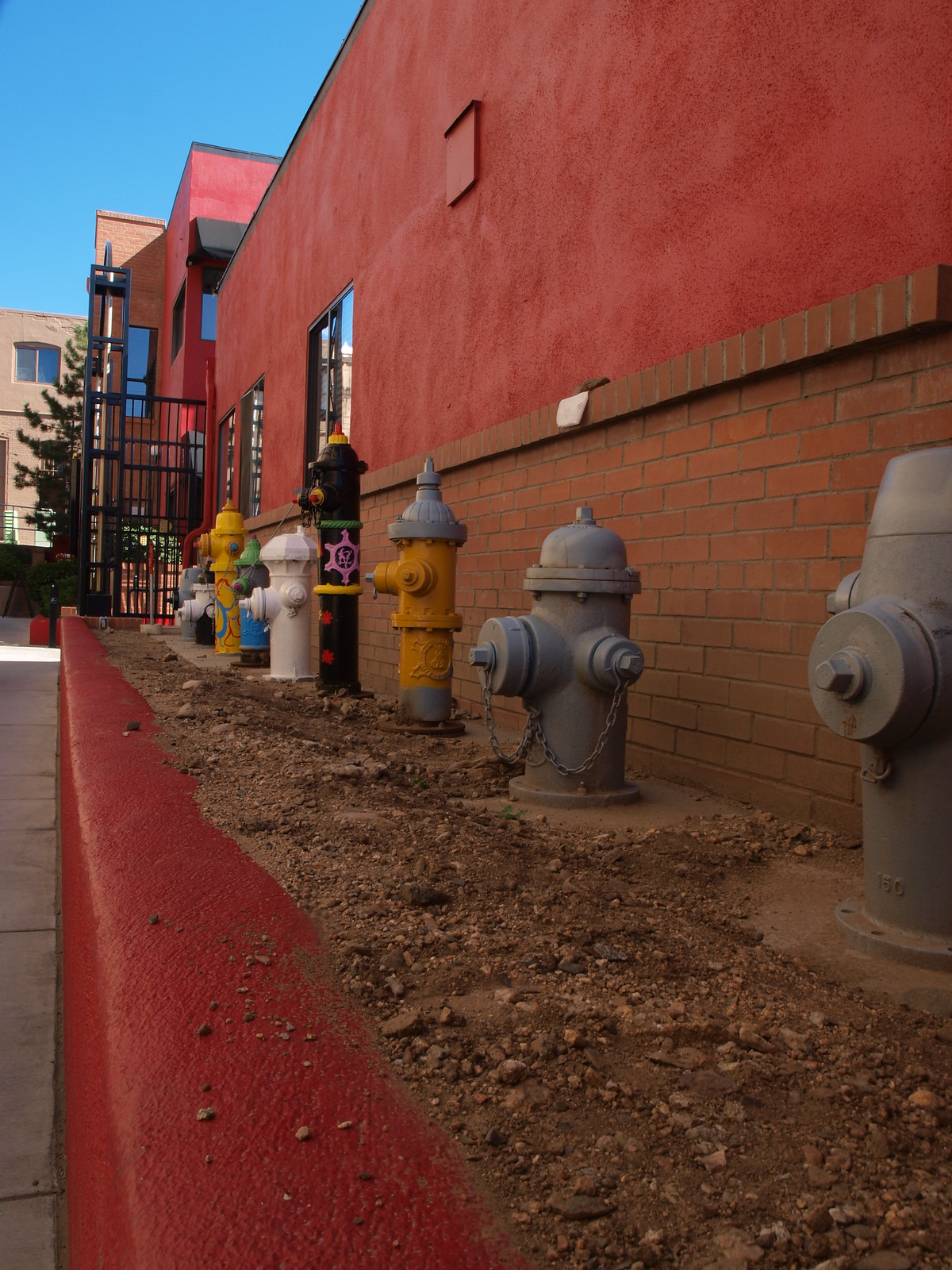This is a detailed color photograph capturing a unique urban scene featuring a display of fire hydrants arranged in a dirt strip against a red brick building. The building's bottom half is composed of reddish bricks, transitioning to a similarly deep red painted upper section, and is adjacent to a sidewalk bordered by a red-painted curb. The strip of soil, flanked by a red-painted concrete edge, holds an assortment of fire hydrants, each buried into the ground, suggesting they are potentially functional.

At the forefront, there are two squat, gray fire hydrants. Following these, there is a sequence of hydrants of varying sizes and vibrant colors: a yellow hydrant with a gray top, a tall black hydrant adorned with pink detailing, a green stripe, and a yellow stripe, a white hydrant, a hydrant with a blue base and a green top, another yellow hydrant with red and blue squiggles, and another white hydrant. There is also mention of a decorative wrought iron gate with an iron tower and a green tree observed towards one side, indicating the image may have been taken in a residential area or near an apartment complex.

The collection of fire hydrants, the red backdrop, and the shadow of a tree create an artistic composition, emphasizing the contrast and variety amidst a shared urban setting.